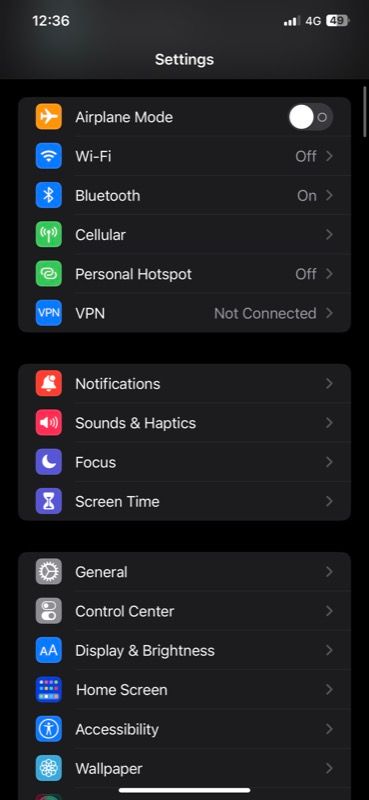The image, captured from a smartphone, displays the device's settings menu. At the top of the screen, the time reads 12:36 PM and the battery is at 49% with the device connected to a 4G network showing three bars of connectivity. The background is a mix of gray and black. 

Central to the image is the word "Settings" in larger font. Listed below it, running from top to bottom on the gray background, are various menu options accompanied by corresponding icons of different colors: 

- **Airplane Mode** (with a toggle switch currently off, displayed by a white button to the left)
- **Wi-Fi** (off, with an arrow pointing right)
- **Bluetooth** (on, indicated by a highlighted icon)
- **Cellular** (an arrow pointing right)
- **Personal Hotspot** (off, arrow pointing right)
- **VPN** (not connected, arrow pointing right)
- **Notifications** (arrow pointing right)
- **Sounds & Haptics** (arrow pointing right)
- **Focus** (arrow pointing right)
- **Screen Time** (arrow pointing right)
- **General** (arrow pointing right)
- **Control Center** (arrow pointing right)
- **Display & Brightness** (arrow pointing right)
- **Home Screen** (arrow pointing right)
- **Accessibility** (arrow pointing right)
- **Wallpaper** (arrow pointing right)

Each setting is represented by an icon of unique colors like orange, blue, green, red, purple, gray, and teal, positioned to the left of the text.